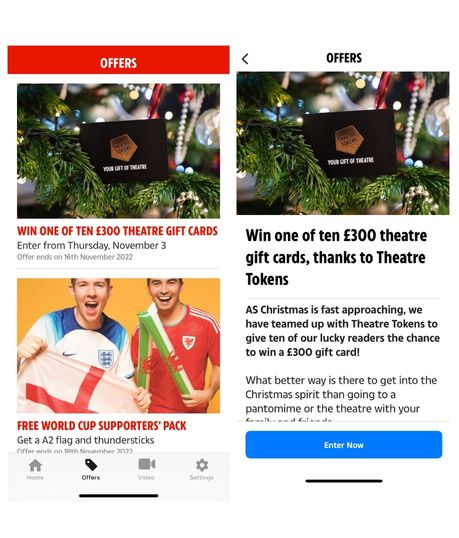This screenshot captures an unknown website with distinct sections highlighting various promotions. 

On the left side, a prominent red banner with the word "Offers" in white lettering draws attention. Below the banner, an inviting image of a black gift card is artfully nestled within the branches of a Christmas tree adorned with strings of pearls and round ornaments. The accompanying text reads: "Win one of 10 £300 theater gift cards. Enter from Thursday, November 3. Offer ends on November 16, 2022."

Further down, there's a joyful image of two young men smiling directly at the camera. The man on the left dons a blue and white jersey featuring a Nike symbol on the left and a blue and white SHIELD symbol on the right, holding a white flag with a red cross. The man on the right wears a red short-sleeved shirt with white stripes on the shoulders and a red and white SHIELD symbol on the right, holding two green and white noise-making sticks. Beneath this image, the text states: "Free World Cup Supporters Pack. Get an A2 flag and Thunder Sticks. Offer ends on November 18, 2022."

On the right side, the word "Offers" appears again, this time in black letters. This section mirrors the left with the same image of the gift card nestled in the Christmas tree. The detailed description reads: "Win one of 10 £300 theater gift cards thanks to theater tokens. As Christmas is fast approaching, we have teamed up with theater tokens to give 10 of our lucky readers the chance to win a £300 gift card. What better way is there to get into the Christmas spirit than going to a pantomime or the theater with your family and friends? Enter now."